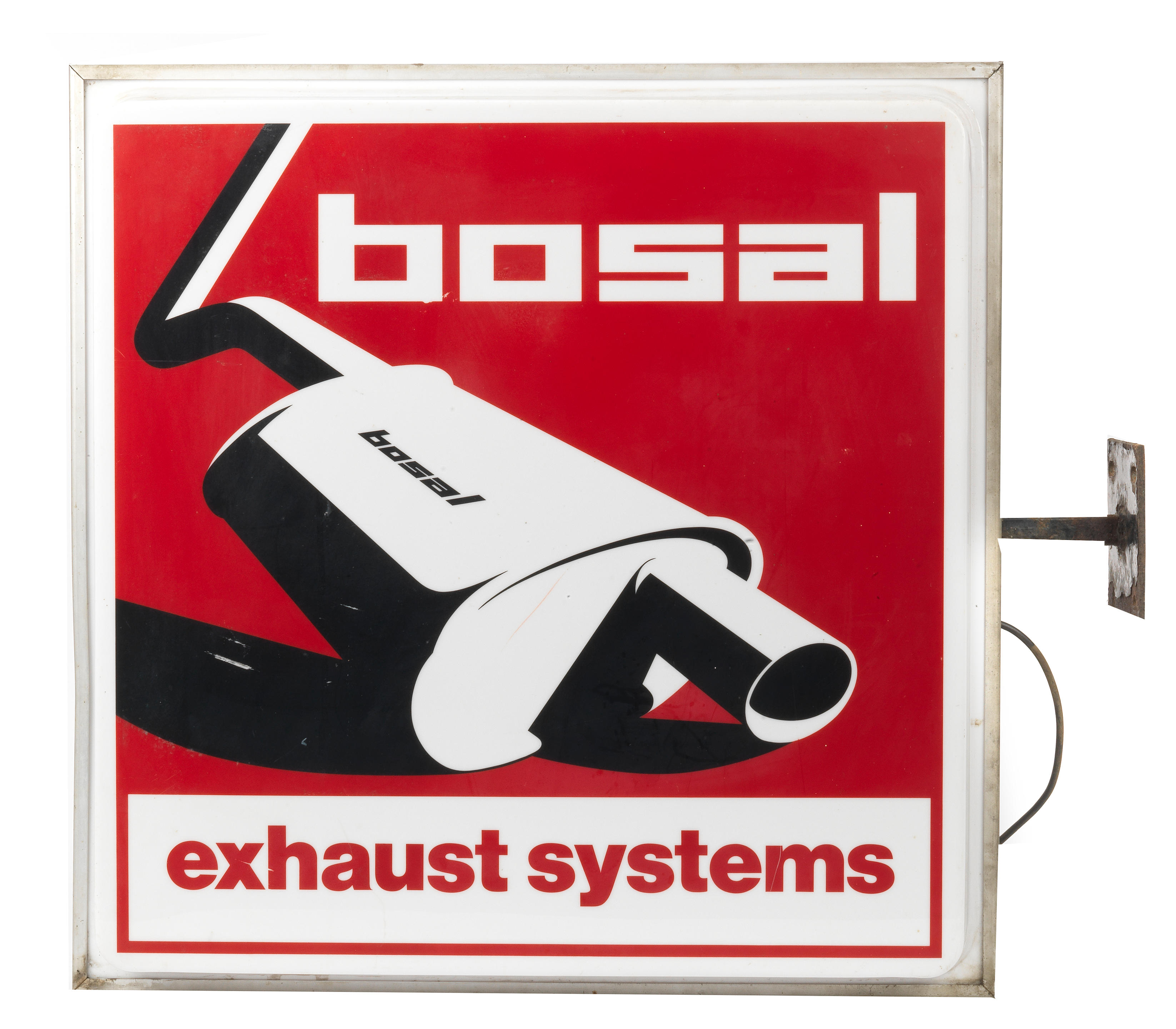This image depicts a square sign advertising "Bosal" exhaust systems. The central design features a large red square with "BOSAL" in block, stylized black letters at the top, and a black-and-white illustration of a muffler right underneath it which also reads "BOSAL." Below the drawing, a white strip with red letters spells out "EXHAUST SYSTEMS." The entire sign is mounted on a white background and supported by a long metal bar extending from the right side, attaching it to the wall via a plate with four brackets. The metal frame and brace appear silver but show signs of wear and chipping. Additionally, a wire or cord is visible, looping out from the bottom right of the sign, suggesting it might be an illuminated advertisement. The overall design is stylized, with a modern yet slightly worn appearance.